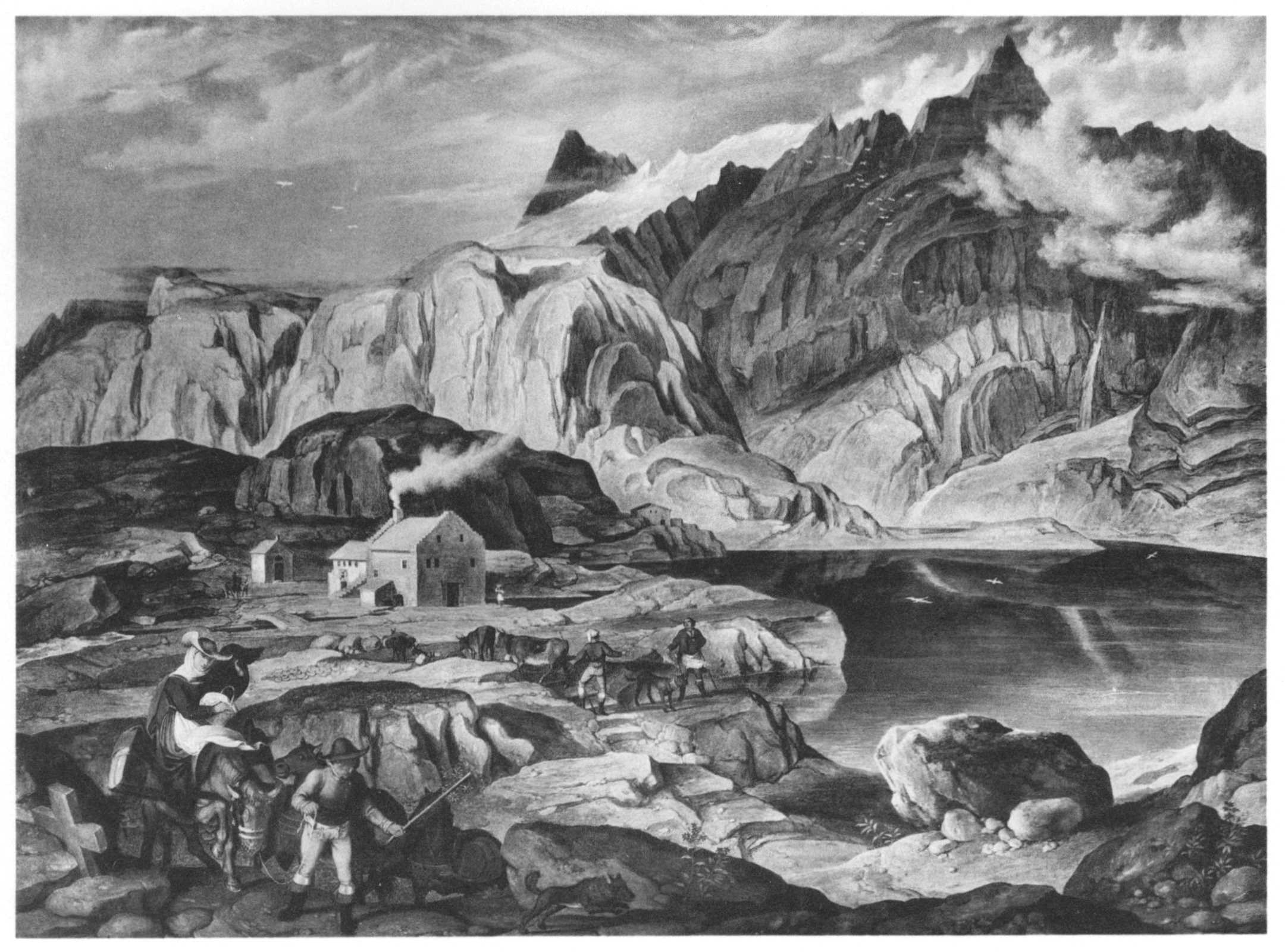This black and white artwork, which could be a charcoal drawing or pen and ink sketch, depicts a historical landscape scene with striking detail. The sky is stormy and filled with dark gray clouds, creating a somber and dramatic atmosphere. In the background, jagged mountain peaks pierce through the cloudy sky, adding to the rugged feel of the scene, while softer, rounder mountains appear closer to the viewer. A lake, or possibly a flattened, watery area, rests at the foot of these mountains, surrounded by a rocky foreground.

In the middle-left of the image stands an old stone house, with smoke billowing from its chimney, suggesting someone is inside, possibly cooking. This house is accompanied by smaller structures that enhance the sense of a lived-in, yet remote and harsh, environment. 

In the foreground, a dynamic scene unfolds with figures engaged in daily activities. A younger boy walks with a stick, followed by a man—possibly his father—riding a horse. This man seems to be guiding the animal carefully over the rocky terrain, perhaps using the stick for stability. Alongside them, a dog runs ahead. Another figure appears to be holding either a young child or a pet while riding an animal, which could be a horse, pony, or donkey. This group is being led by another man, who looks down to navigate the rugged path. Small nondescript figures in the background add layers of depth to this intricate composition. 

Overall, the intricate interplay of figures, animals, and the rugged landscape captures a moment steeped in history and the harsh beauty of a bygone era.